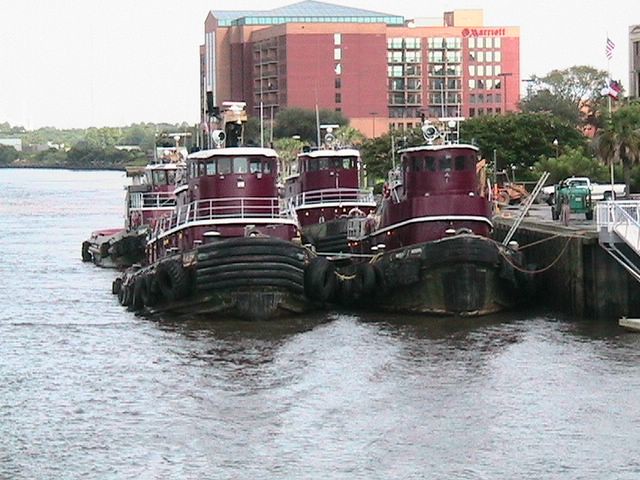In this image, four maroon-colored tugboats with black bottoms are docked along a cement pier to the right. Each tugboat is equipped with large black tires hanging from the sides and reinforced rubber bumpers in the front. The boats feature white-trimmed windows, white roof accents, and white railings, providing a uniform appearance. Some variations exist, such as the upper level of one boat missing the white fence.

To the left of the dock, there is an open body of water, extending to a distant tree line. Central in the background, behind the tugboats, stands a tall hotel with a peachy-pink facade displaying the "Marriott" logo in red at the top right. The hotel has numerous windows, suggesting it is a multi-story building, possibly around 10 stories high.

Adjacent to the dock in the right corner of the image, a flagpole stands beside a white pickup truck parked near some construction equipment. The scene is further framed by an abundance of trees, enhancing the sense of a bustling, waterside area.